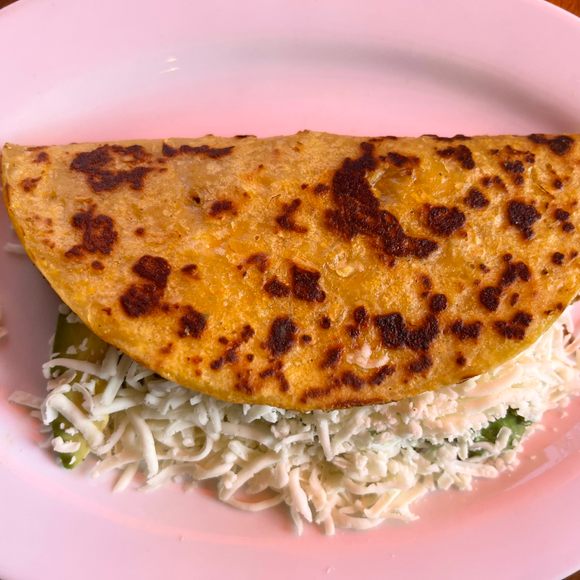This color photograph features a close-up of a golden brown, hard-shelled taco placed on its side on a pink plate that occupies the entire frame. The taco appears to have been fried or pan-fried, with visible toasty brown marks and black specks on its crispy shell. The interior is partially obscured, but spilling out from the edges is a mound of white shredded cheese, not yet melted, and a couple of green avocado slices. The taco’s texture and coloration suggest it has cheddar cheese grilled onto its outer shell, adding an extra layer of crispiness and flavor. The focus on the food, with just small segments of the plate visible in the top left, top right, and bottom right corners, draws the viewer's eye to the detailed textures and colors of this appetizing dish.